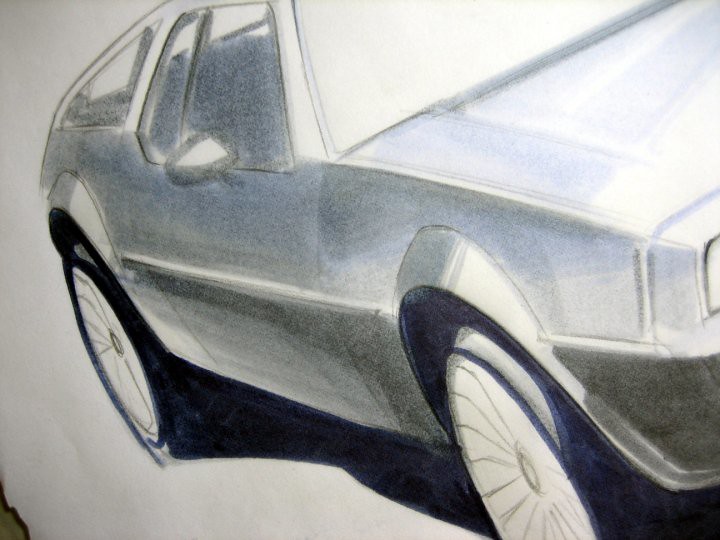A detailed, hand-drawn sketch of a DeLorean is depicted with remarkable precision in black, white, and shades of gray. The car, recognized for its iconic role in "Back to the Future," is shown in its unmodified, original form without the movie's distinctive modifications. This two-seater features characteristic elements like the small triangle windows and sleek, silvery body, achieved possibly through silver pencil or detailed shading to enhance its reflective surface. Notably, the focus of the image is on the right side of the car, particularly the wheels, but from our perspective, it's the left side of the photo, along with one of the rearview mirrors situated just left of the center. The rims are intriguingly depicted as though they were made of paper, giving a unique twist to the otherwise highly realistic portrayal. The windows display a hint of transparency, suggesting details within the car, such as where a license plate might be. Subtle blue tints outline the wheels, adding depth and interest to the sketch, which otherwise remains text-free.